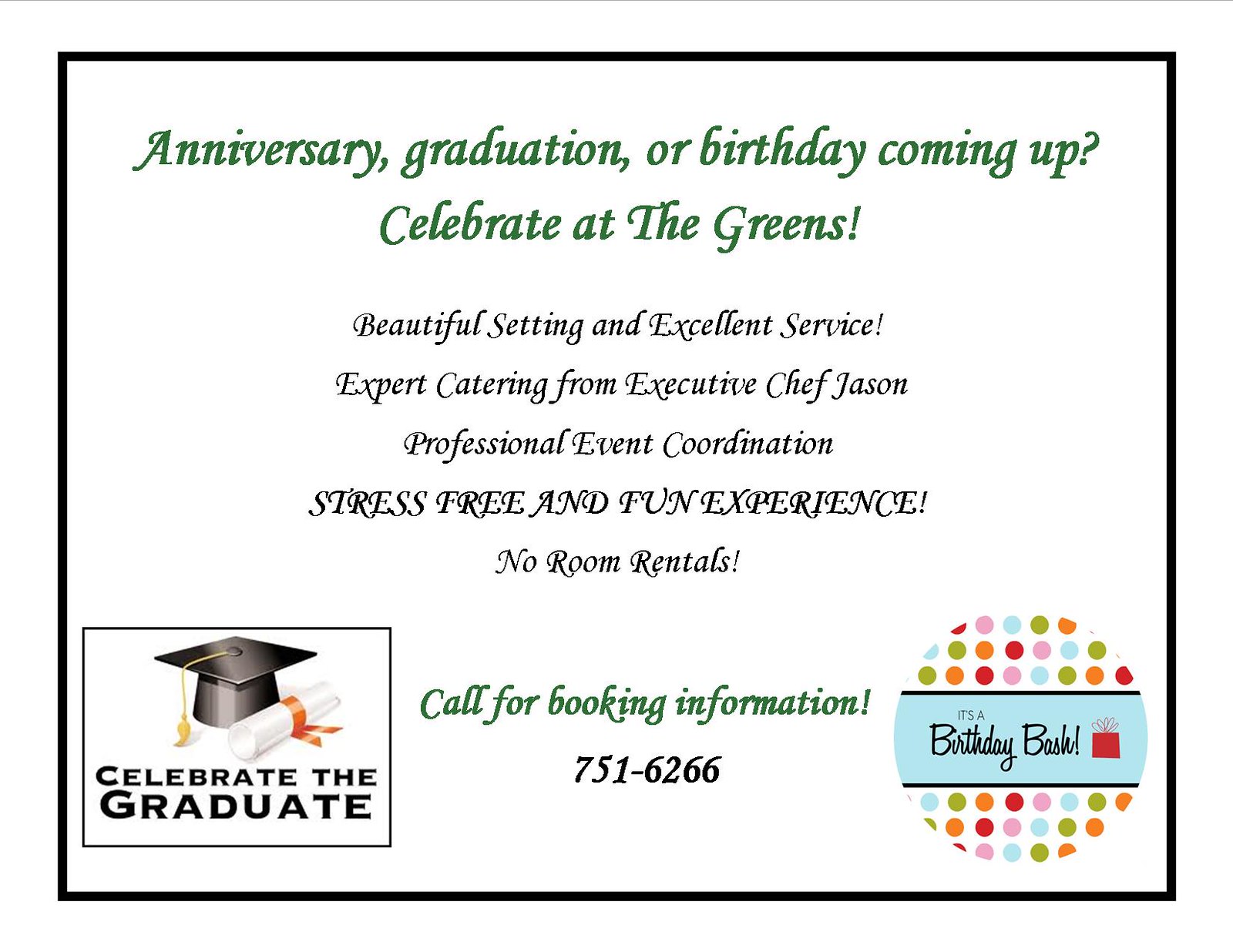This is an advertisement set against a white background, featuring a colorful polka dot design overlay. At the top, bold green text reads: "Anniversary, Graduation, or Birthday Coming Up? Celebrate at The Greens!" Beneath this, smaller black text details the offerings: "Beautiful Setting and Excellent Service. Expert Catering from Executive Chef Jason. Professional Event Coordination. Stress-Free and Fun Experience. No Room Rentals." 

In the lower left corner, there's a bordered square displaying an image of a graduation cap, diploma, and tassel, captioned "Celebrate the Graduate." Centrally placed, green text invites readers to "Call for Booking Information" with the phone number 751-6266 in black below. On the right-hand side, a small circle features the words "Birthday Bash" in black text on a blue background, alongside a red cake illustration. The whole design is vibrant and engaging, perfect for catching the eye and enticing potential customers.